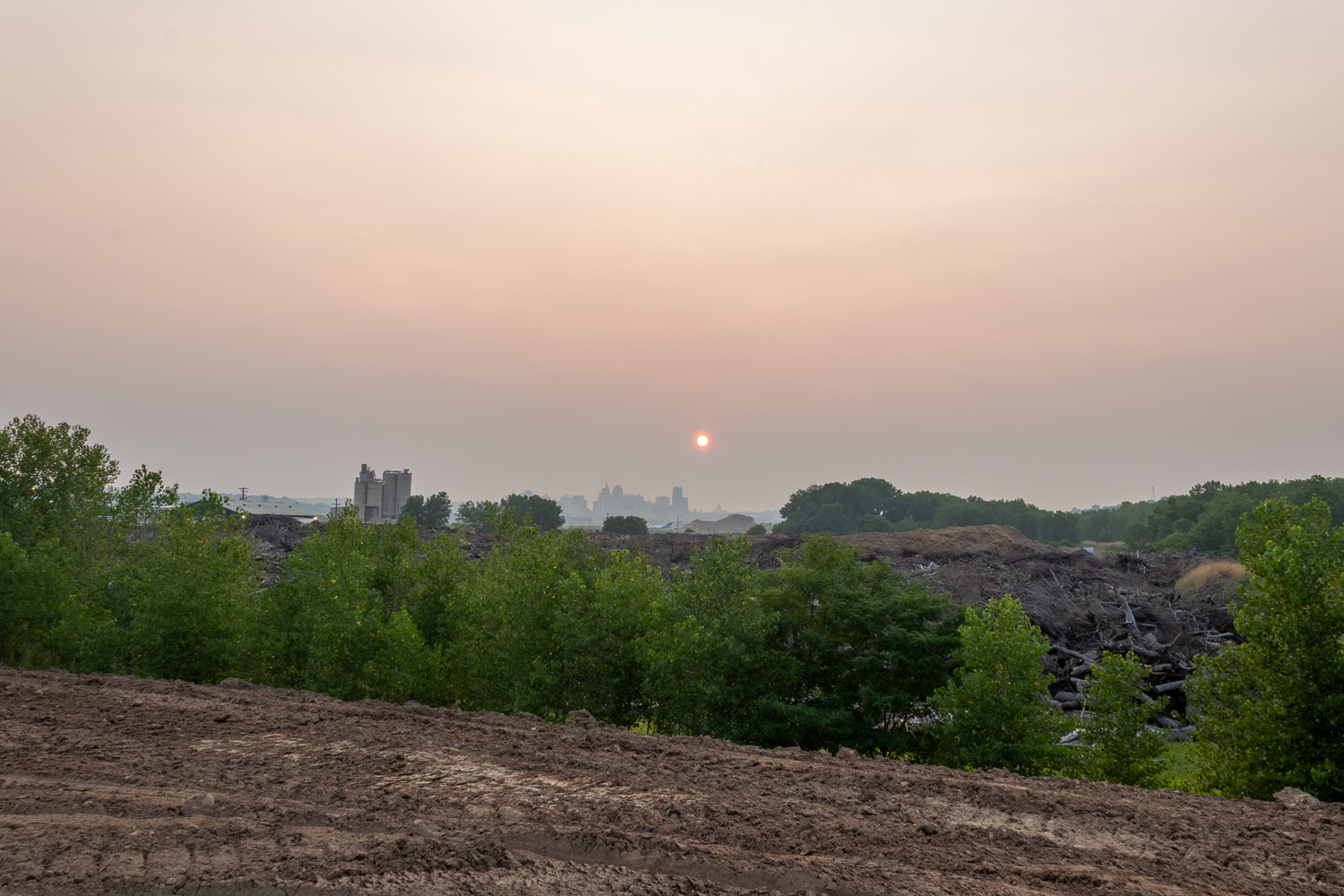This landscape-oriented photograph captures an outdoor scene dominated by natural and human elements. In the foreground, a clearing of brown soil and mud is marked with visible tractor tire tracks. Beyond this, a small ravine is lined with scattered green trees and bushes. Further back, a barren area appears, populated sparsely with dark, dry trees and debris that suggest the remnants of tree-cutting or a fire. Past this desolate stretch, another line of vibrant green trees marks the boundary before the scene transitions to an urban backdrop.

On the horizon, the silhouettes of tall industrial buildings and a hazy city skyline can be seen. The sky above is strikingly divided into hues of blue and reddish-orange, indicative of a setting sun. The sun itself is a small, amber-colored circle, adding a warm glow to the sky. The image is bright and clear, taken during the daytime with ample natural light, and showcases a mixture of natural and industrial landscapes under a vivid sunset.